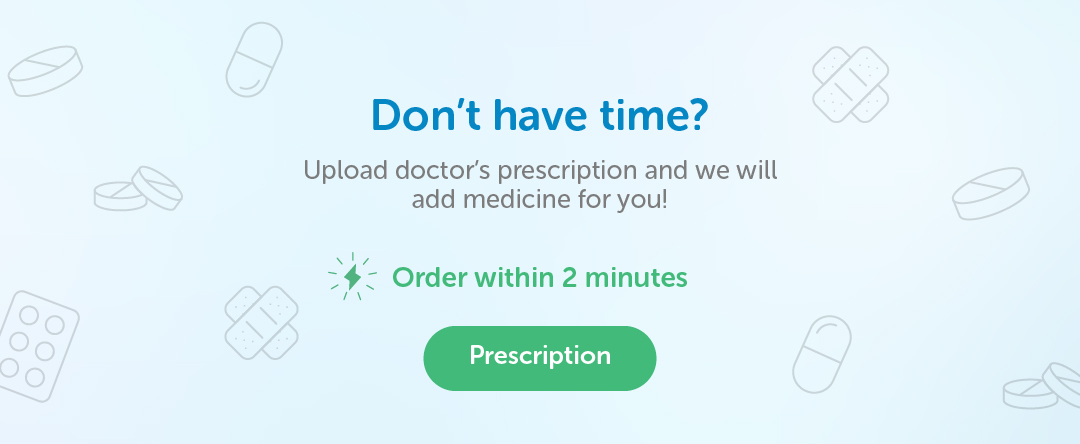The image showcases a webpage promoting a convenient prescription upload service. The main text on the page reads, "Don't have time? Upload your doctor's prescription and we will add the medicine for you. Order within two minutes." This prominent message is designed to guide users quickly through the prescription submission process. The background features a light blue gradient, adding to the calm and trustworthy feel of the page. Scattered across the backdrop are graphic designs of pills in various colors like blue, green, and grey, subtly reinforcing the medical theme. The overall aesthetic is clean and professional, aiming to streamline the user's experience with minimal effort.